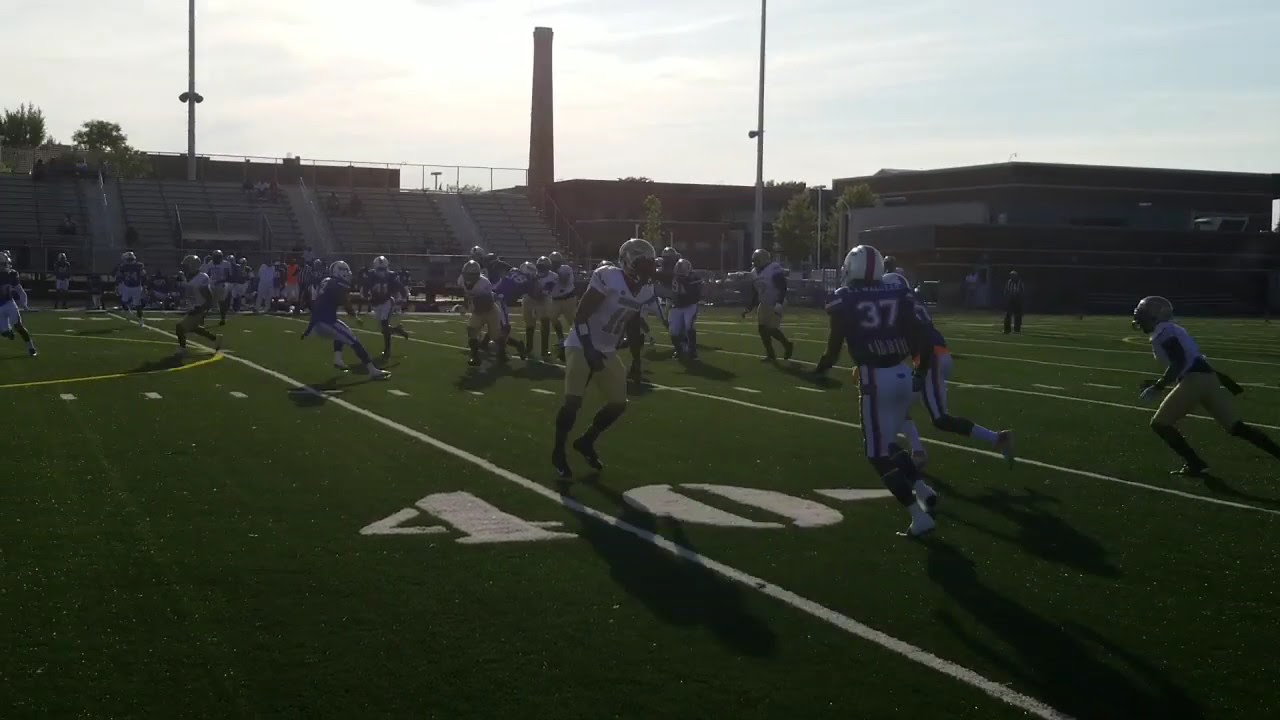The photograph captures an intense moment of a high school football game in progress on an AstroTurf field. It shows two teams—one in blue jerseys with white pants and the other in white jerseys with yellow pants and gold trim. Prominent numbers visible are 37 and 16, with the players positioned around the 35 or 40-yard line. The action appears to be happening mid-play, highlighting a player with number 37 running toward the center while an opposing player converges on him. Surrounding the field are medium-sized bleachers, tall lighting poles, and a grayish-blue sky with scattered clouds. In the background, there are various buildings, possibly including a school and an industrial-looking structure with a smokestack, suggesting an urban or suburban setting. The field is also bordered by some trees, and the scene is bathed in soft sunlight, casting shadows of the players on the ground.